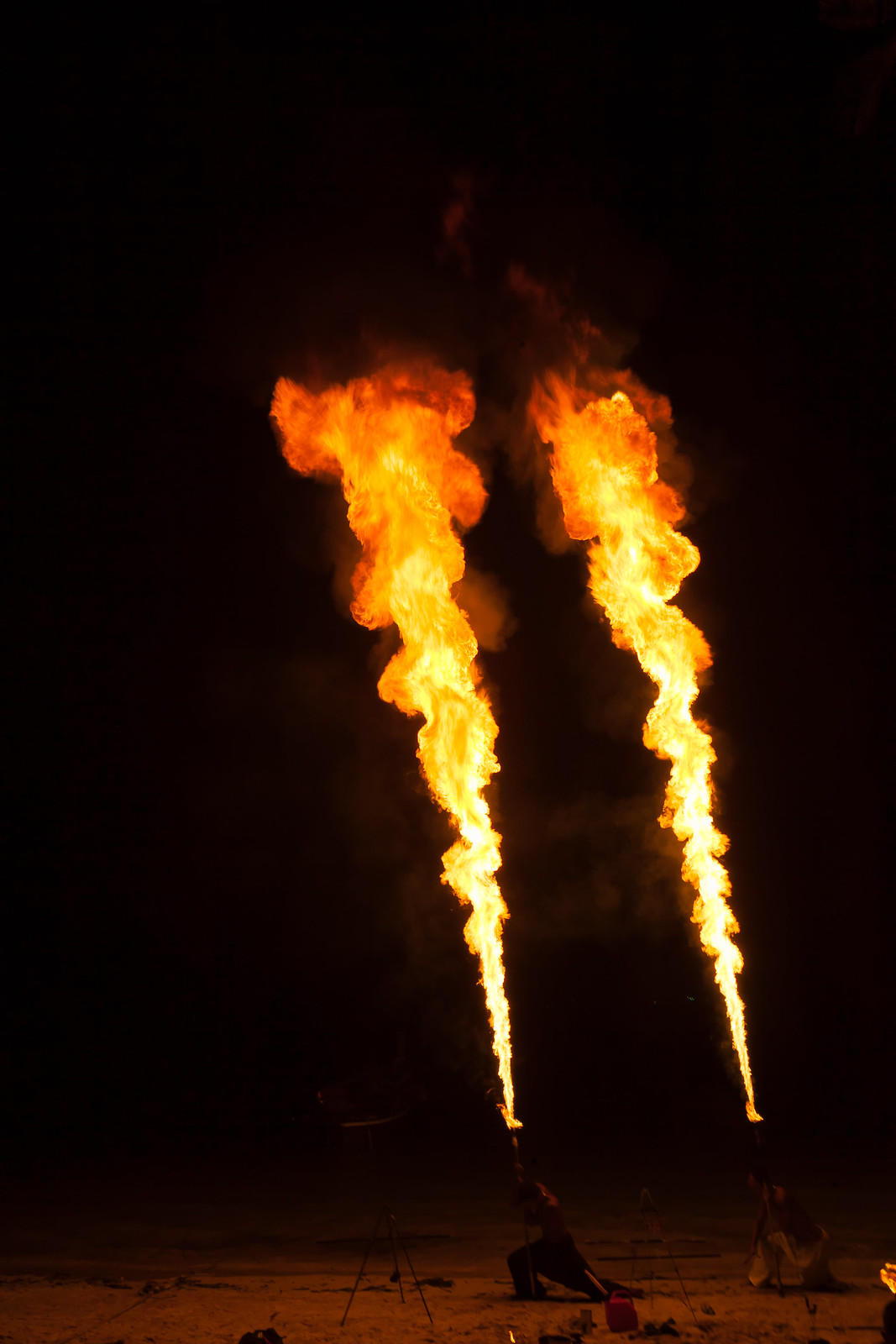In this striking nighttime photograph, two men, kneeling side by side about five to 10 feet apart, are in the midst of an impressive fire performance, presumably in a desolate area resembling a desert or dirt-covered ground. Each man holds a flamethrower in their right hand, with massive, dragon-like gouts of fire shooting high into the dark sky. The flames, initially narrow at the base, expand and become more intense and orange as they rise. Their performance area is dimly illuminated by the fire, revealing what appears to be concrete flooring or a street setting and even a red gas can on the ground nearby. The atmospheric darkness adds to the drama, making the fiery display the central focus, with the flames brilliantly illuminating the otherwise invisible surroundings.